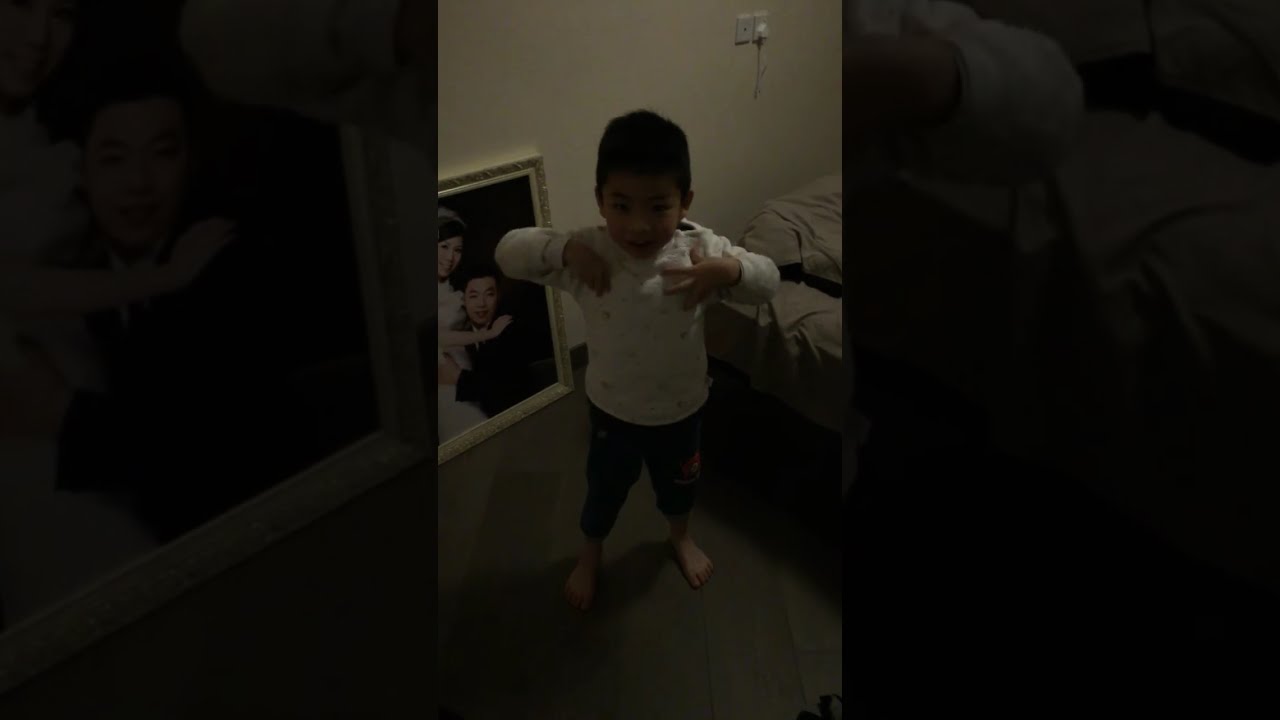The photo captures a young boy with short brown hair, wearing a white long-sleeve shirt and dark-colored pajama pants, standing barefoot in a bedroom. He is looking up at the camera and smiling, with his hands resting on his shoulders. The room has white walls, tiled flooring, and features a bed with white sheets and a white pillow to the right of the boy. To the left, there's a framed picture with a black background, depicting a bride and groom hugging, possibly the boy’s parents, in a white frame. The room also contains a white outlet and a switch plate on the wall.